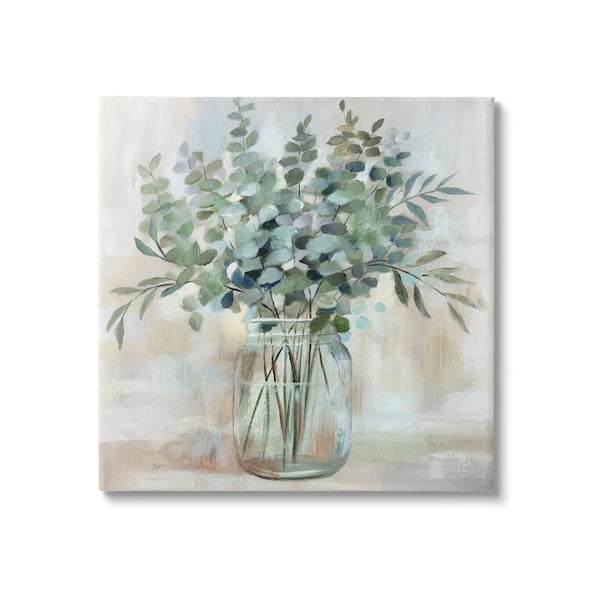This detailed painting features a clear glass vase or jar, reminiscent of a mason jar, filled with an array of green leaves, with no flowers present. The leaves vary in shape and size—some are round, some slender and cylindrical, while others are jagged. The stems are visible through the water in the vase, accentuating its transparent quality. The background is a muted, textured off-white or cream with hints of light brown and blue-beige, creating a blurred, ombre effect. The artwork, characterized by its matte finish and short, cohesive brushstrokes, emphasizes the natural greenery against the understated backdrop.